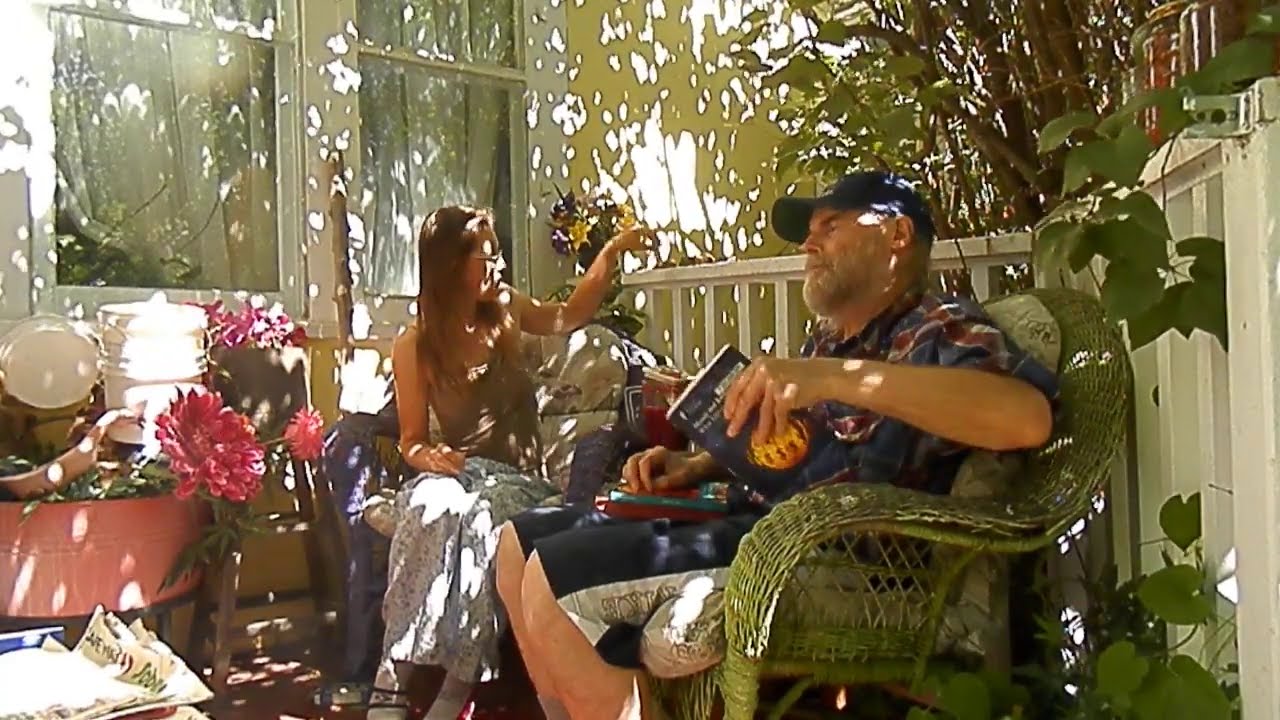In this image, a couple is relaxing on their vibrant and flora-filled porch, bathed in dappled sunlight filtering through a lush canopy of trees. The man, seated in a green wicker chair with a white outdoor pillow, appears to be in his 40s. He sports a beard, a navy blue baseball cap, and a blue and red flannel shirt paired with black and white shorts. He holds a blue and yellow book in his left hand, with additional books in his lap, their spines showing turquoise and red hues. The woman beside him, sitting in a purple wicker chair, wears glasses, a dark green tank top, and white pants. Her long blonde hair cascades over her shoulders, and she points behind her toward the garden past the white wooden railing. The cozy scene is complemented by abundant flowers and outdoor equipment such as buckets and a salmon-colored basin to the left of the woman. The background showcases their charming house with yellow walls, white-framed windows, and a scattering of light spots that create a warm and inviting atmosphere.